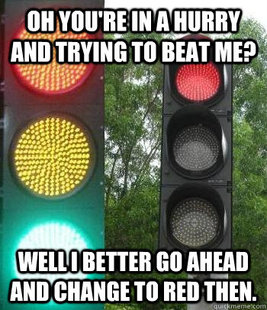In the image, a bald, muscular man with a short beard and a hairy chest is at the center, wearing only underwear that doesn't fully cover his buttocks. He is posed on a bed on his fists and knees, with a cylindrical black and white pillow beneath him. Behind him lie several black pillows, and the bed features a red, gray, black, and white camouflage-patterned throw. The bed is framed by two elongated posts and a dark wood-stained headboard. The room's walls are painted a muted dark gray. Written at the bottom of the image in white Impact font with a black outline is the word "Hai." The overall color scheme of the image includes brown, blue, black, white, peach, tan, red, and gray, typical of meme-style presentation.